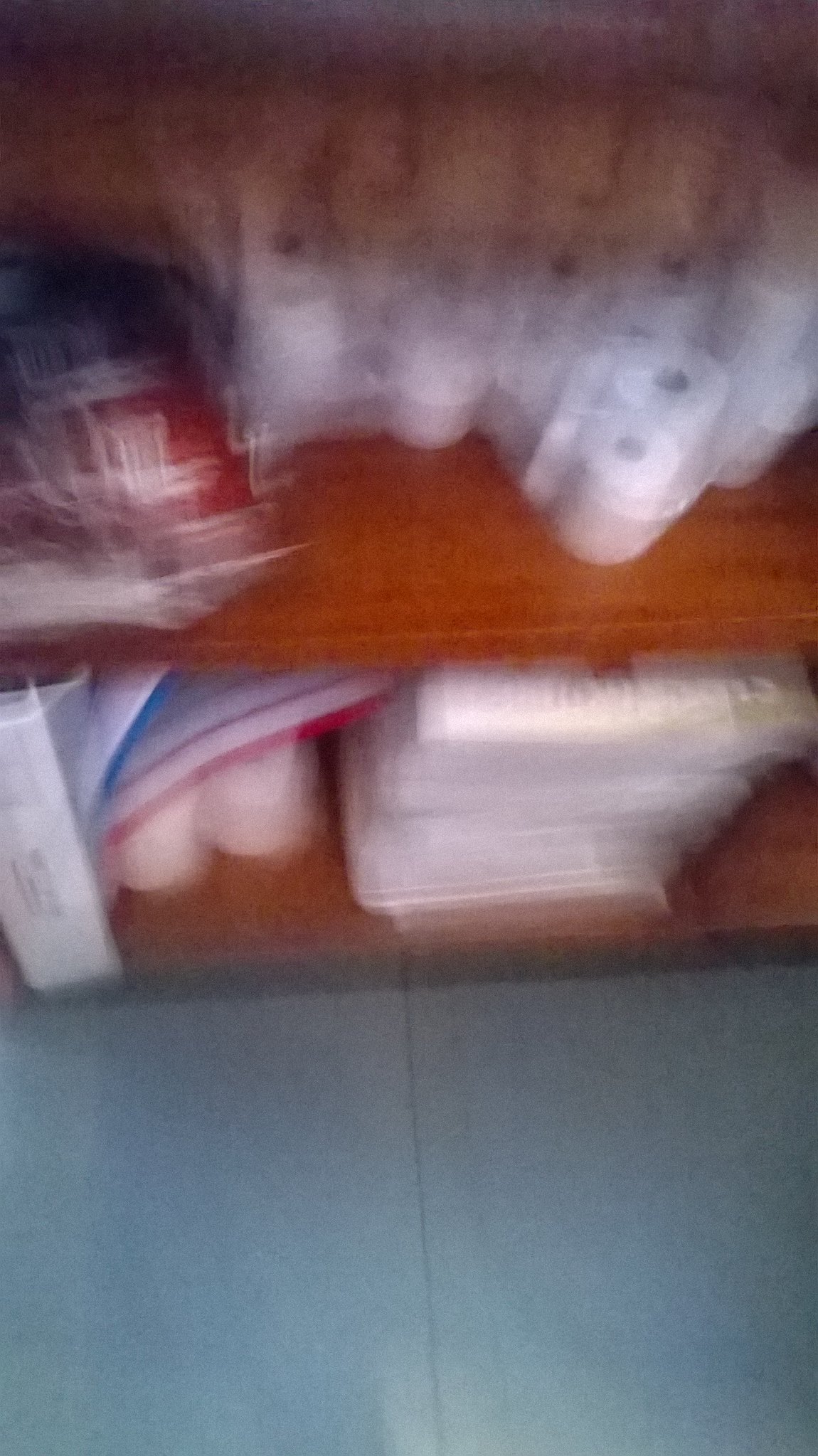The image showcases a close-up of two wooden shelves, each filled with different items. 

On the bottom shelf, there is a stack of white magazines neatly placed next to a three-ring binder situated on the left side. Additionally, there is a red and white striped item that could be a poster or cloth draped on this level.

The top shelf, although significantly blurry, appears to hold several rolls of white material that could be either toilet paper or receipt paper. These rolls extend towards the back of the shelf. Situated on the left, there is some kind of packaging containing red items that resemble pouches.

Though certain details are indistinct due to the blurriness of the image, the overall composition and arrangement of the items are evident.